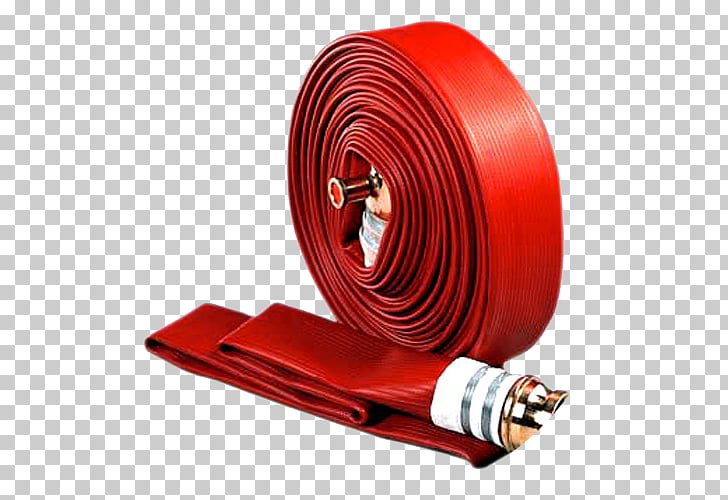The image depicts a neatly coiled, vintage-style red fire hose against a white and gray checkered background that indicates image transparency, typical of stock photos. The background is rectangular and aligned horizontally. Dominating the center of the image, the fire hose is wound around a spool with a visible metal attachment at the spool's core. In front of the standing roll is a folded section of the same hose, showcasing its distinct features. This folded portion has a white cylindrical collar and a metal spout designed for water discharge. Additionally, there is a metallic piece at the end of the fold and another piece attached to the spool's center, adding functional details to the hose’s appearance. The fire hose occupies less than half of the image, leaving the checkered background unobstructed. There are no other objects, text, or people present in the image, emphasizing the focus on the fire hose itself.